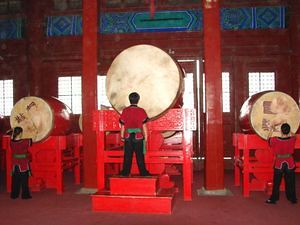This image depicts a vibrant indoor scene, likely in an Asian country, featuring three individuals engaged in a drumming performance. The focal point is a set of three large drums, positioned in a row upon red, wooden platforms that vary in height. Each drum stands on a wooden stand, with two medium-sized drums flanking a significantly larger central drum. The drum faces are covered with what appears to be worn, stretched leather, while the drums themselves are red.

The performers, two girls and one boy, all dressed in red jackets and black pants, are positioned in front of the drums. The boy, situated in the center, stands on a two-step riser to reach the massive central drum. The girls stand by the medium-sized drums, positioned to the left and right. The room is awash in red hues, from the risers and columns to the walls, creating a bold backdrop for the performance. 

Above the drummers, the upper part of the walls features blue geometric designs, possibly part of wallpaper or painted decor, and there are windows and windowed doors with glass panels. The environment appears to be a traditional wooden building, enhancing the cultural ambiance of the scene.